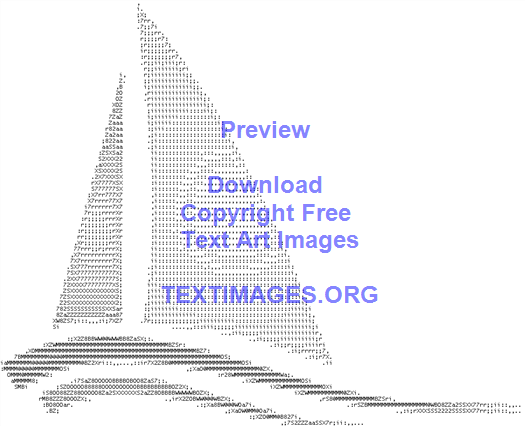This image features a simplistic, text-based illustration of a sailboat against a white background. The sailboat is constructed from black characters arranged to form different shading patterns. The boat comprises four distinct parts: a small, darker sail on the left, a larger, lighter sail on the right, and two curved dark waves underneath that mimic the boat's hull and the surrounding water. Overlaid centrally on the sailboat in blue text are the words: "Preview," followed by a row of spaces, then "Download," "Copyright-Free," "Text Art Images," and finally, "www.textimages.org." The unique feature of the image is its text-based creation, indicating that the entire sailboat and accompanying waves are rendered solely using various text characters.